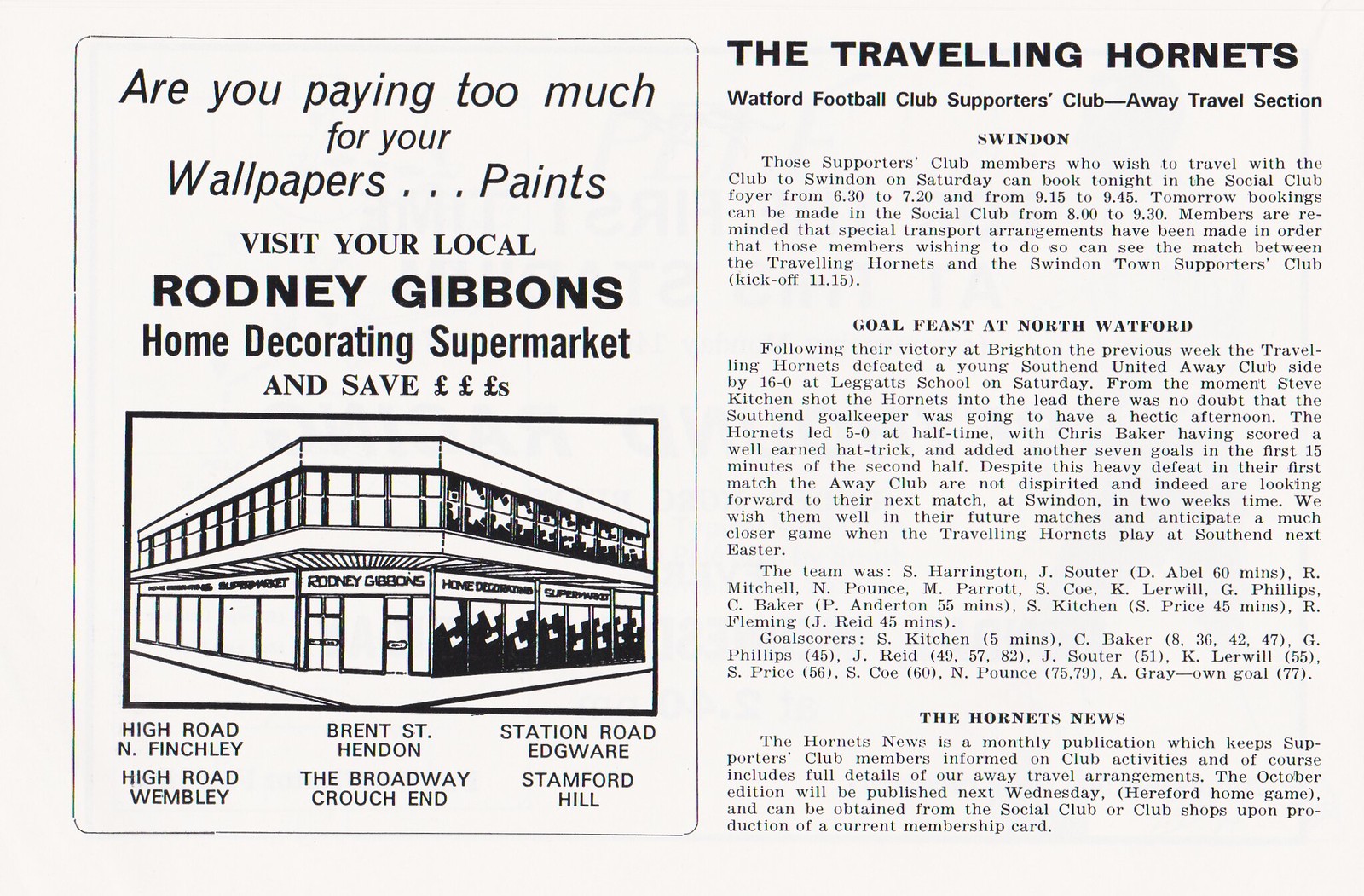The image features a vertically oriented page with a white background and black print. On the left side is an advertisement for Rodney Gibbons Home Decorating Supermarket, featuring a drawing of a Rodney Gibbons building inside a square. The advertisement asks, "Are you paying too much for your wallpapers, paints? Visit your local Rodney Gibbons Home Decorating Supermarket and save pounds, pounds, pounds."

On the right side, there is an article titled "The Traveling Hornets Watford Football Club Supporters Club Away Travel Section." The article is divided into three sections, each with separate text underneath them. The sections are labeled "Swindon," "Goal Feast at North Watford," and "The Hornets News."